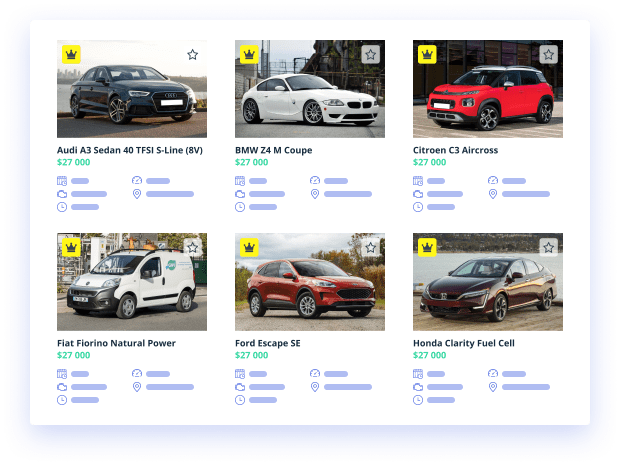Here is a cleaned-up and detailed caption for the image described:

---

This screenshot displays an app or website dedicated to selling cars, showcasing six vehicle listings. Each listing features a vehicle image accompanied by relevant details. Notably, all six images have a yellow square icon with a black crown in the upper left-hand corner, and a clickable star in the upper right-hand corner to mark the vehicle as a favorite.

In the top row:

1. The first image is of a black Audi A3 Sedan, 40 TFSI S-Line EV, priced at $27,000.
2. The second image shows a white BMW Z4 M Coupe, also priced at $27,000.
3. The third image features a red Citroen C3 Aircross with a black roof, for $27,000.

In the bottom row:

4. The first image is of a white Fiat Forino Natural Power van with black accents, selling for $27,000.
5. The next image shows an orange Ford Escape SE, a compact SUV crossover, with a price tag of $27,000.
6. The final image displays a maroon Honda Clarity Fuel Cell, priced at $27,000.

Each listing offers potential buyers a visually distinct option to consider.